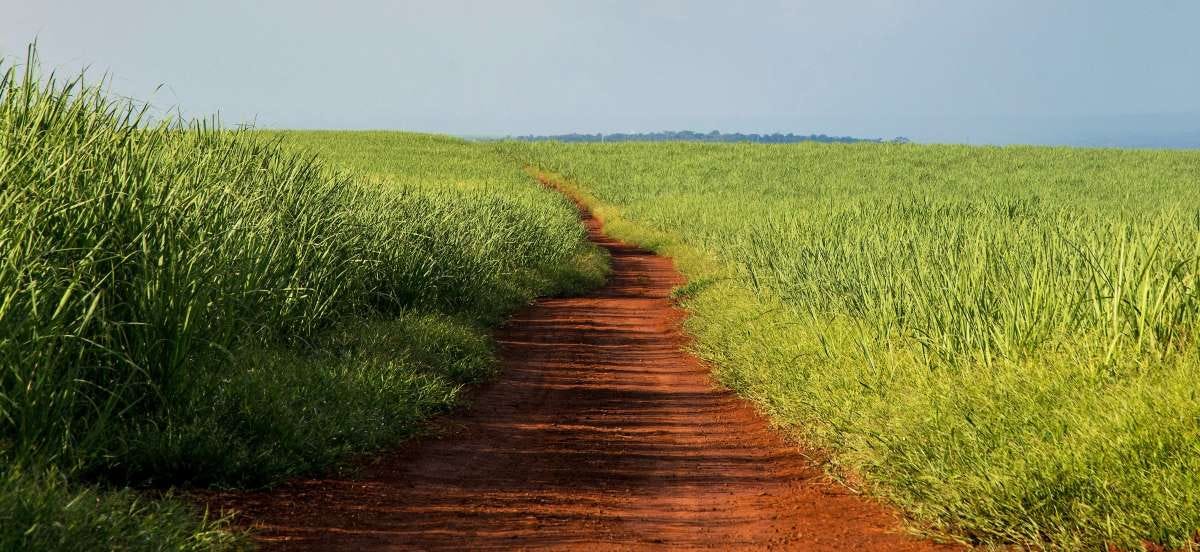The image depicts a serene countryside scene featuring a central dirt path bisecting expansive fields of tall grass under a clear, light blue sky. The path, approximately three to four feet wide, starts at the bottom center of the image and extends vertically, becoming wider as it proceeds into the distance. On either side of the path, the grass transitions from a lighter, sunlit green on the right to a darker, shadowed green on the left. The horizon is marked by a distant tree line, with the trees forming a dark, blurry silhouette against the sky. The top part of the image is dominated by a cloudless sky that shifts from a whitish-blue on the left to a medium blue on the right, suggesting a bright, clear day. The overall composition suggests a point-of-view perspective of someone standing on a tranquil walking path, capturing the peaceful and sprawling beauty of the countryside.